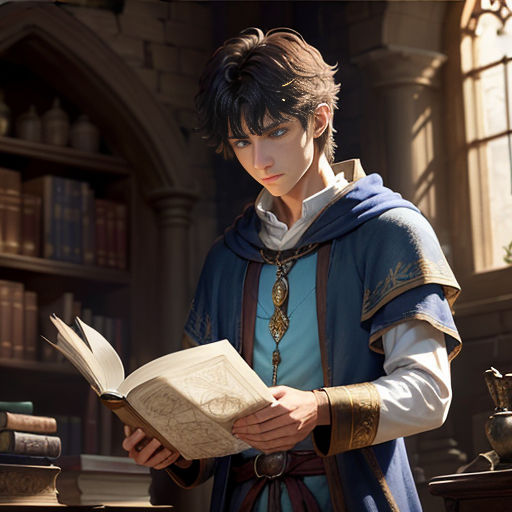This detailed image appears to be a stylized, almost computer-generated, artwork reminiscent of Final Fantasy, depicting a young, white-skinned man in his early 20s with cross-eyed brown hair that is slightly long and unkempt. He is standing in what looks like a castle library, with brick walls and a bookcase behind him filled with encyclopedias and history books. The young man is dressed in an elaborate, two-toned robe, light blue and dark blue, tied with a belt, and beneath it, he wears a high-collared white shirt. He also has a prominent gold necklace around his neck. The light shining through a grid-patterned window highlights the scene, casting shadows around him. He is holding an intricate book with geographical drawings, lost in concentration as he gazes down at its pages.